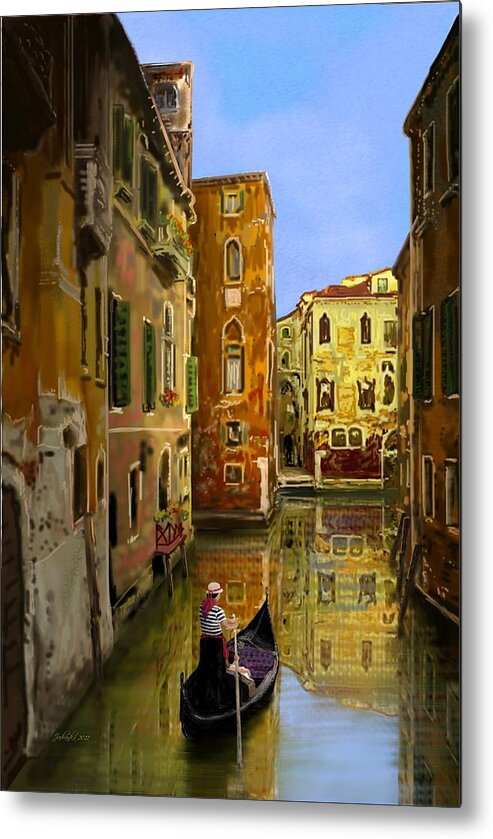This image depicts a serene painting of a gondolier navigating the narrow canals of Venice with at least one passenger onboard. The gondolier, dressed in a white and navy striped shirt, dark pants, and a red scarf, wears a straw hat as he uses a long pole to propel the gondola through the calm water. The scene captures the charm of Venice's old, somewhat ornate buildings, painted in varying shades of brown and terracotta. One of the edifices has a peculiar melting effect, possibly due to the artist's choice of soft, low-contrast colors, reminiscent of a gentle digital filter. Tall and adorned with multiple windows, the structures on either side of the canal are beautifully reflected on the water's surface. The gondolier faces away from the viewer, guiding his boat along what feels like the city's picturesque back alleys, contributing to the painting's overall tranquil and picturesque atmosphere.